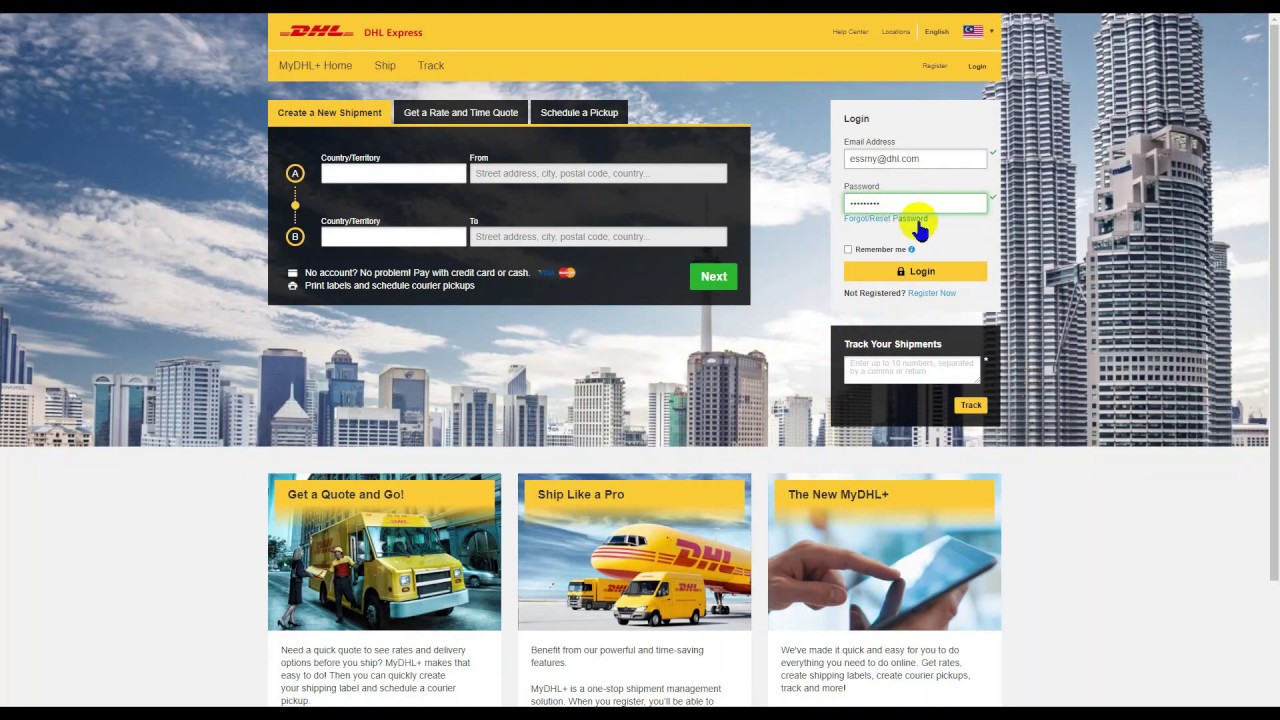This image is a screenshot from the DHL Express website, displaying the "My DHL Plus Home" page. The top section features a yellowish-orange rectangular header with tabs for "Ship" and "Track." On the right side of the header, there is a flag with stripes and a blue field containing a crescent moon and a star, next to the language selection indicated as "English."

The main background of the image showcases a picturesque cityscape under a bright blue sky dotted with fluffy white clouds. Prominent, round, and tall buildings occupy the left side of the image, appearing closer to the viewer, while additional large buildings extend into the distance, creating depth.

Central elements of the webpage include rectangular sections where users can "Create a New Shipment," "Get a Rate and Time Quote," or "Schedule a Pickup." There's also a login area for users to enter their email address and password. At the bottom of the screen, additional options to "Get a Quote" and "Ship Like a Pro" are emphasized, promoting the new features of My DHL.